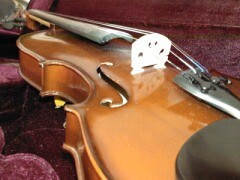This image features a close-up view of a violin, captured from one end to the other, lying horizontally. The violin, with its brown body and curved edges, is remarkably shiny, reflecting the light that illuminates it. A distinctive silver bar spans its surface, while black padding is visible at the head of the instrument. The violin is depicted with strings prominently stretching across its body.

The instrument rests on a reddish burgundy or purple-pinkish fabric, potentially a rug or carpet, or even inside a cushioned case. This background fabric enhances the visual appeal of the scene with its rich color tone. Though there are some indistinguishable objects behind this fabric, the focus remains clearly on the violin itself.

Overall, the detailed capture highlights the glossy and polished appearance of the violin, its intricate parts, and the ambient setting, making the musical instrument stand out.